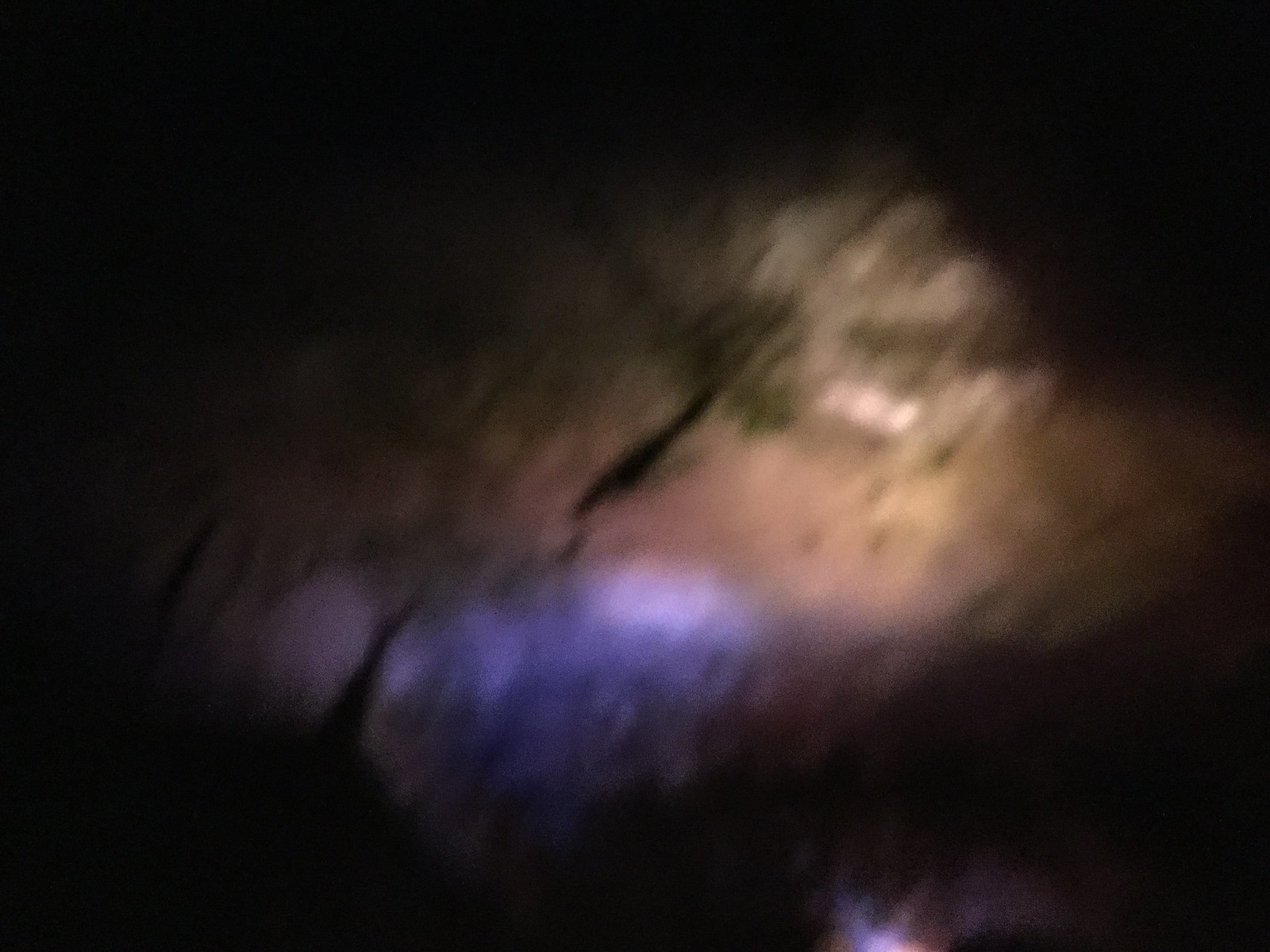The image presents an extremely out-of-focus scene that evokes the experience of driving at night, with the faint suggestion of trees and branches. Predominantly shrouded in black, the image features a conspicuous, illuminated area that serves as the primary focus. In the lower right corner, bursts of color – including purples, reds, and browns – stand out against the dark backdrop. The blurred foreground is a swirl of various shades: blues, purples, light blue, tan, brown, yellow, green, light green, white, and black. It vaguely resembles a tree trunk or limb, possibly illuminated by vehicle headlights. However, due to the lack of clarity, the exact nature of the scene remains uncertain.